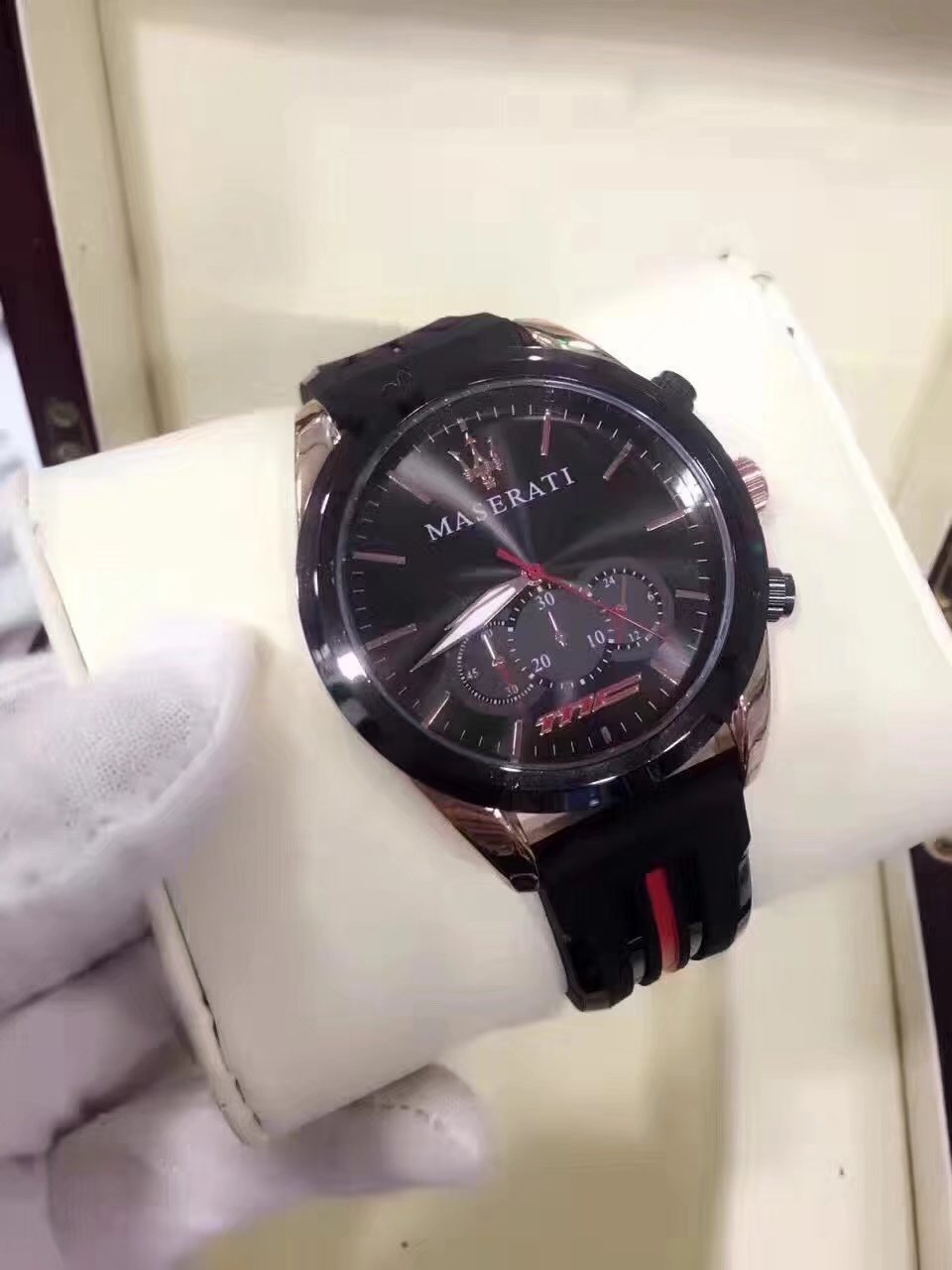The image showcases a sophisticated black band watch from the renowned brand Maserati. The watch features a striking black face with the brand name "Maserati" elegantly displayed in white font on the upper portion. At the bottom of the face, the initials "MC" are prominently highlighted in a vibrant red font. The hour and minute hands are white, while the second hand stands out in red, adding a subtle yet striking contrast. Both the watch face and the band are predominantly black, with a distinctive red stripe running down the center of the band, enhancing its stylish appeal. The watch is luxuriously presented on a pristine white cushion, typical of those found in high-end watch shops. A seller's hand, adorned with a crisp white glove, is visible in the image, suggesting a poised presentation to a potential buyer. The overall setup exudes a sense of elegance and refinement, indicative of a premium product offering.